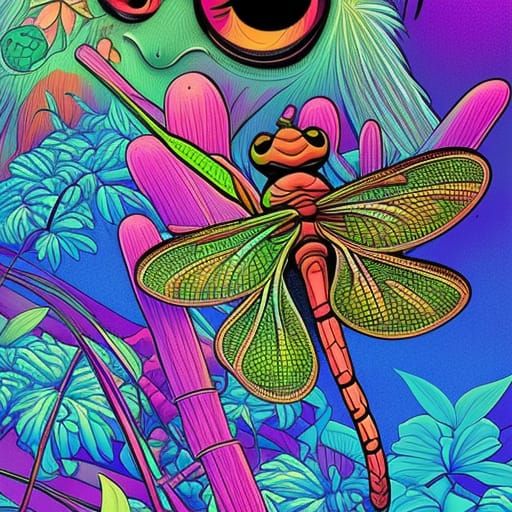The image is a psychedelic, cartoonish digital artwork depicting a vibrant dragonfly. The dragonfly, viewed from above, features a pinkish-orange segmented body and two sets of bright green wings. It has large, prominent black eyes and appears to be flying amidst teal-colored vegetation and blue and pink flowers. The background is predominantly blue with patches of bright neon colors including pink, orange, and mauve. Additionally, there's a light green creature with furry hair and big, moon-shaped orange and pink eyes partially hidden behind the foliage, adding to the surreal atmosphere of the scene. The overall effect of the image is highly detailed and vividly colorful, emphasizing a psychedelic aesthetic.